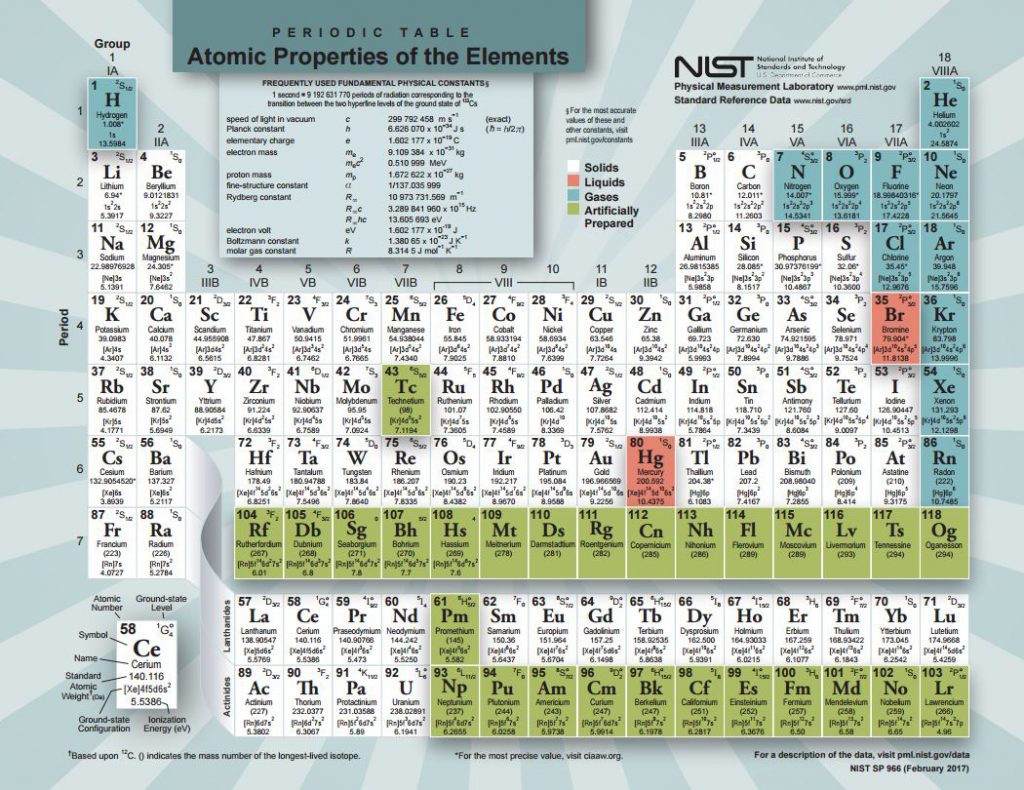Presented here is a poster by the National Institute of Standards and Technology depicting the periodic table of elements. The chart meticulously details the atomic properties of each element, categorized by distinct color groups. Elements are arranged traditionally, beginning with hydrogen and helium at the top, and progressing to the more radioactive elements displayed in green at the bottom. The periodic table features elements grouped in blue, white, green, and red, providing a visual representation that enhances the understanding of the elemental organization and classifications.